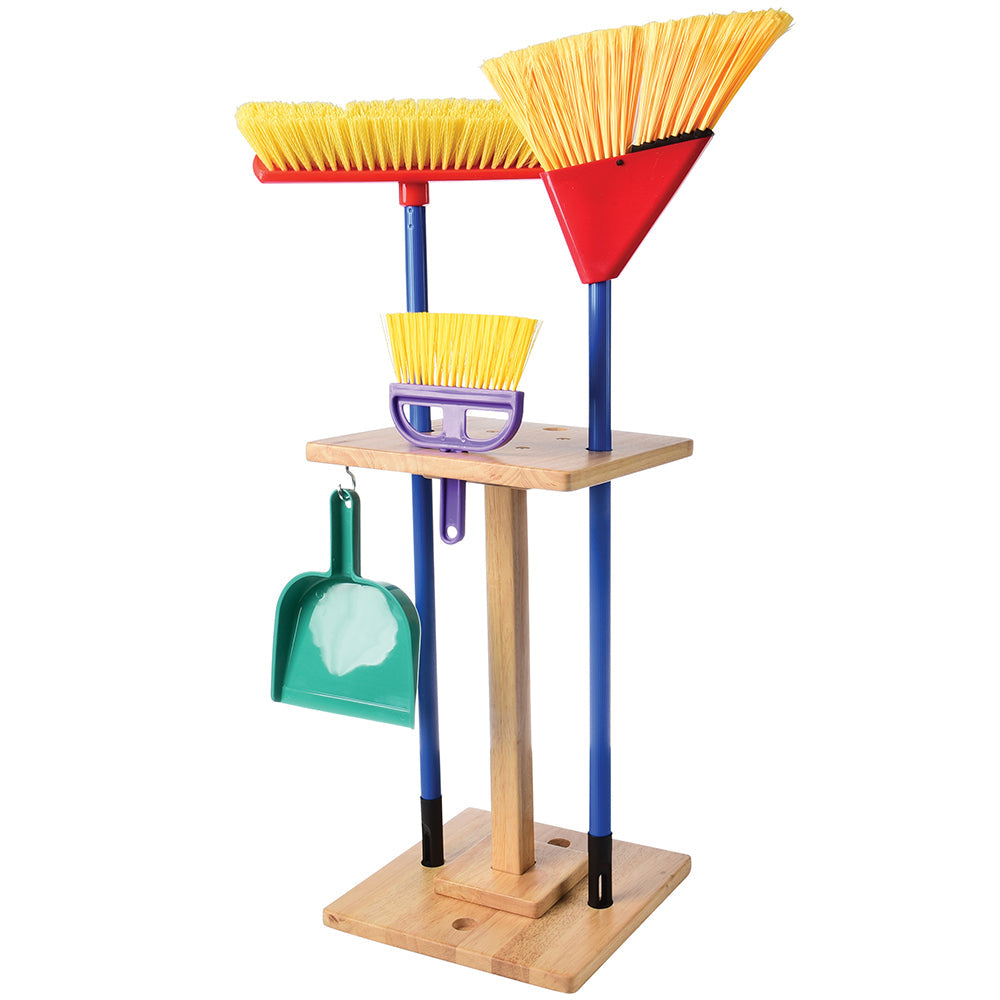The photograph depicts a meticulously crafted wooden cleaning organization stand, set on a square brown wood base. This stand features a central squared pole connecting to another square platform with multiple holes designed to securely hold various cleaning supplies. On the side of the stand, a green plastic dustpan hangs from a metal U-shaped hook via a hole in its handle. The stand showcases three different types of brooms: a small purple-handled hand broom with yellow bristles, a triangular broom with a blue handle and yellow bristles, and another broom with similar features. The primary colors within the image include shades of light brown, green, blue, purple, and yellow, set against a white backdrop. The overall arrangement emphasizes both functionality and aesthetic organization of house cleaning tools.